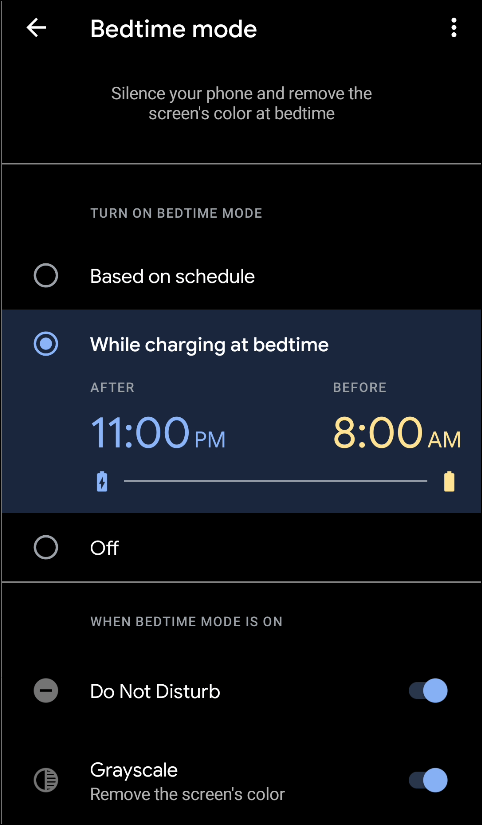This vertical image, likely from a smart device, features a sleek user interface with a solid black background devoid of any texture or dimension. In the upper left corner, a white arrow points to the left. Adjacent to it, "Bedtime mode" is prominently displayed in bold white text, accompanied by an icon of three vertical dots signifying additional options. Below, in a softer, almost gray text, instructions read: "Silence your phone and remove the screen's color at bedtime."

A thin, horizontal line segments the display. Below this divider, the option "Turn on bedtime mode" is presented in the same soft gray font. The interface showcases two main choices: "Based on schedule" (currently not selected) and "While charging at bedtime," boldly highlighted in white and selected.

Details of the bedtime settings reveal a blue time indicator for "After 11 p.m." and a yellow indicator for "Before 8 a.m." These times are connected by a line with a battery icon—initially adorned with a lightning bolt and transitioning to another battery icon in yellow, indicating fully charged status.

An unselected "Off" option follows, separated by another line. Further down, beneath the header "When bedtime mode is on," the option "Do Not Disturb" is toggled on, depicted in blue, along with "Grayscale," which is also toggled on, actively removing the screen's color to aid in improving sleep habits.